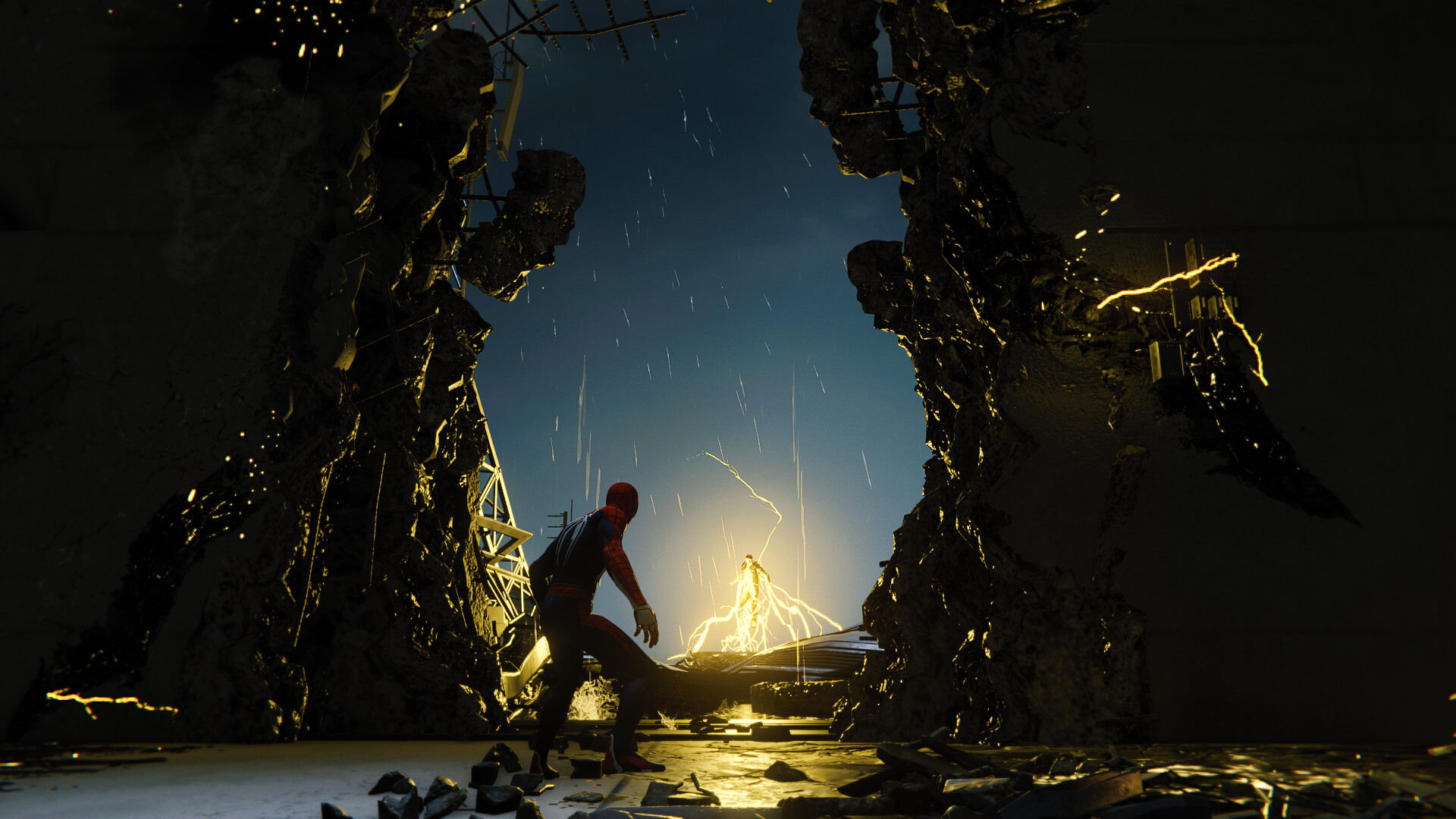The vivid photograph, possibly a still from a video game or a scene from "The Amazing Spider-Man 2," showcases a dramatic, action-packed moment. In the foreground, a figure clad in a blue and red suit, resembling Spider-Man, stands intently, his gaze fixed on something in the distant night. He is within a cave-like structure with rocky surfaces around him and an opening leading to an outside vista where the sky is painted dark blue with streaks of lightning. A ladder is visible at the cave's entrance. The night scene is illuminated by the crackling sparks from a villainous figure, likely Electro, who floats in the background surrounded by glowing yellow electricity. The structure, with its damaged walls and joined metal pieces at the top, suggests a building that's been ravaged by a fierce battle, adding to the scene's intensity and suspense.